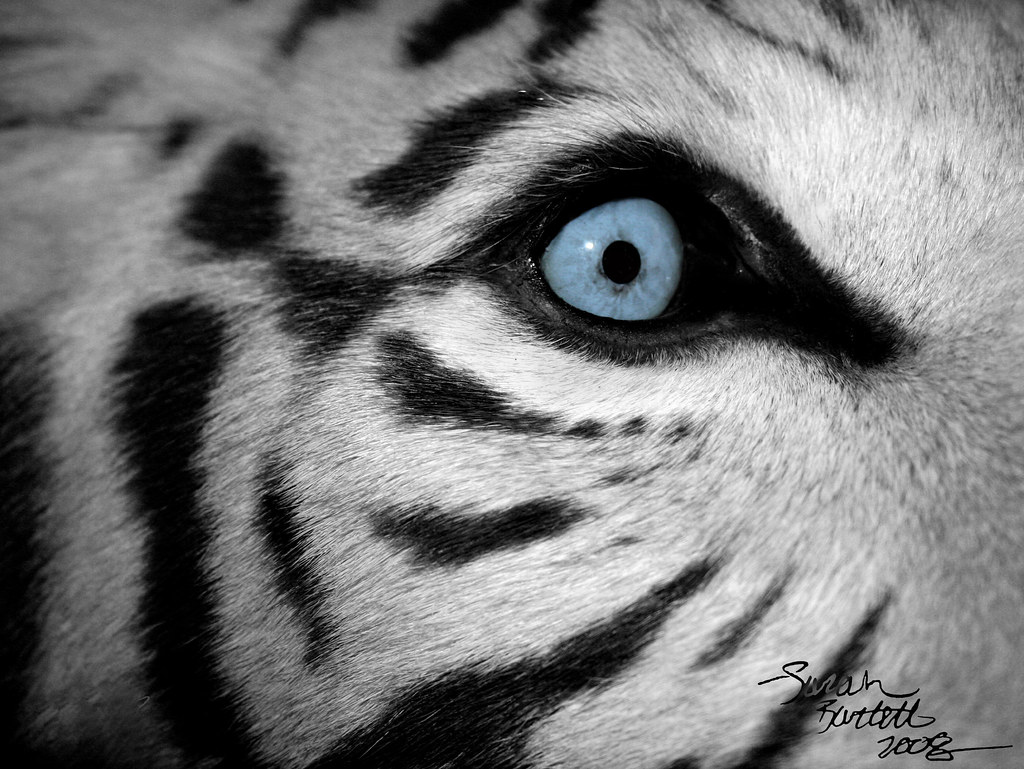This image features an extreme close-up of a white tiger's eye, with the eye itself serving as the focal point. The bright blue iris, punctuated by a solid black pupil, commands immediate attention. Surrounding the eye, the fur is predominantly white, accented by a few black stripes. A small area of black skin lies just around the eye. The framing of the image shows a hint of fur to the right, a minimal amount above, slightly more below, and a bit to the left of the eye, with no visible ears or nose. The eye is positioned in the lower-left section of the upper right quadrant of the image. At the very bottom, a cursive signature reads "Sarah Bartlett 2008" across three lines.